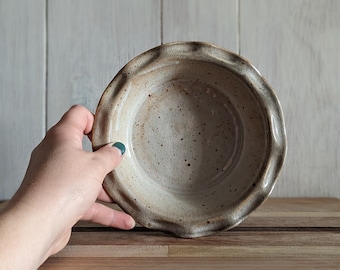A photograph showcases a woman's hand, adorned with green nail polish, delicately holding a small, handmade clay bowl on its side to reveal its interior. The bowl, roughly the size of her hand, has a beige hue reminiscent of lightly cooked pie crust and is speckled with brown dots, suggestive of its handcrafted origin. The bowl’s surface is marked with the characteristic indentations of pottery that was thrown by hand, featuring rivets around its somewhat deep edges. This scene unfolds against a rustic backdrop of shiplap siding and wooden planks, evoking a farmhouse aesthetic, while the bowl subtly contrasts with the grayish tones of the wall behind.